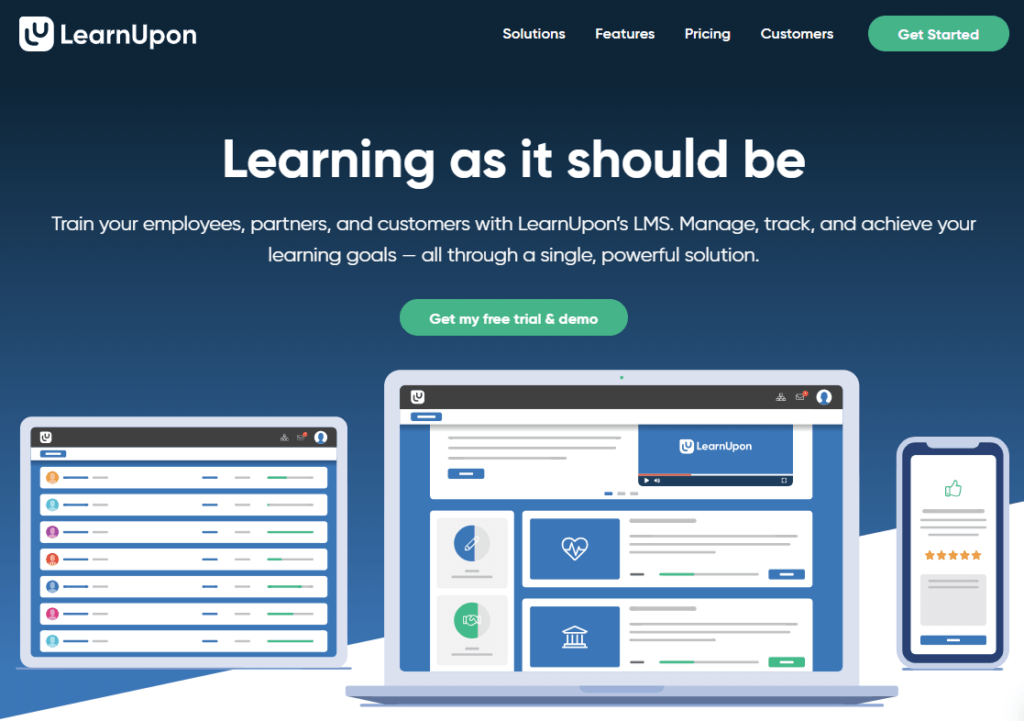This image displays the homepage of LearnUpon's website, set against a gradient blue background that darkens towards the top and lightens towards the bottom. The LearnUpon logo, featuring a white "U" and an L-shaped design, is prominently displayed. The website header includes clickable features such as "Solutions," "Features," "Pricing," "Customers," and a green, rounded "Get Started" button.

Central to the page is a bold white text declaration: "Learning as it should be." This is followed by a brief overview: "Train your employees, partners, and customers with LearnUpon's LMS. Manage, track, and achieve your learning goals all through a single powerful solution." Below this text, another green, rounded button labelled "Get My Free Trial and Demo" invites user interaction.

The bottom section of the page showcases images of various devices displaying different parts of the LearnUpon website. A central laptop screen exhibits the main LearnUpon interface, predominantly blue and white with some green elements. To the left, a monitor screen presents a different aspect of the website, featuring white bars with colored icons and supplementary text. Additionally, an image of a smartphone illustrates another webpage with a five-star rating, a green thumbs-up icon at the top, and a blue bar at the bottom.